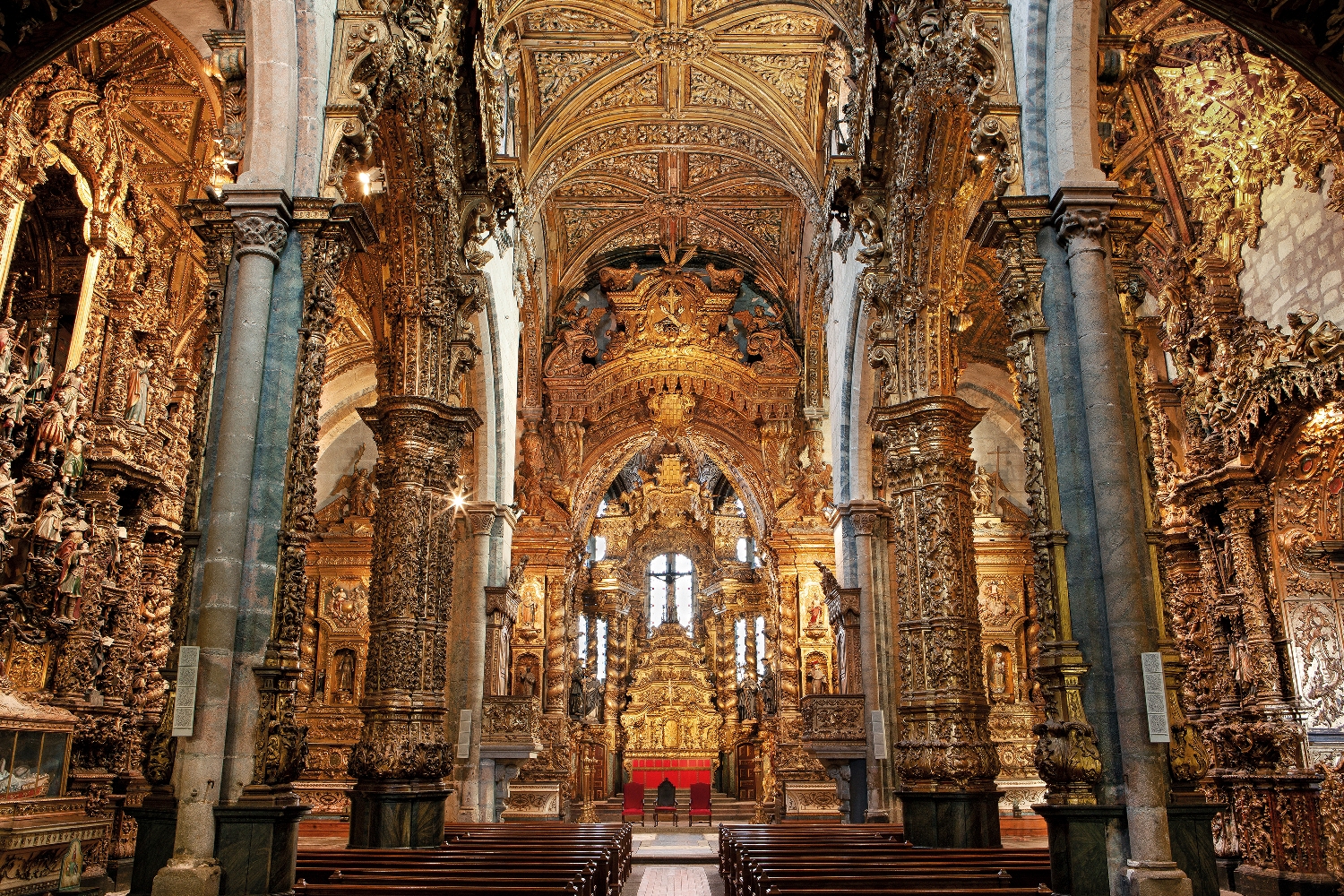This photograph captures the interior of an extraordinarily ornate cathedral, likely designed in Baroque or Rococo style. The vantage point is from the back of the sanctuary, revealing an expansive view down the central aisle towards the main altar. The structure is supported by towering pillars on either side, constructed from light sandstone gray or concrete, with intricate detailing. The vaulted ceilings above the nave are lavishly decorated, predominantly with gold and yellow embellishments.

To our immediate left and right, grand arches frame additional altars that are richly adorned with figurines, beams, and crosses, all predominantly gold in color. The wooden pews, displayed in rows along both sides of the aisle, are dark and polished, contrasting with the opulent surroundings. Walls adorned with meticulously carved wooden panels enhance the visual richness with embedded images and floral patterns.

At the front of the cathedral, the main altar stands as a focal point, draped with a vibrant red cloth. Three chairs, also upholstered in red fabric, are arranged centrally in front of the altar, with a crucifix subtly discernible in the distance. Despite the absence of people in the photograph, the sheer detail and extravagant decoration convey the sanctity and grandeur of the space.